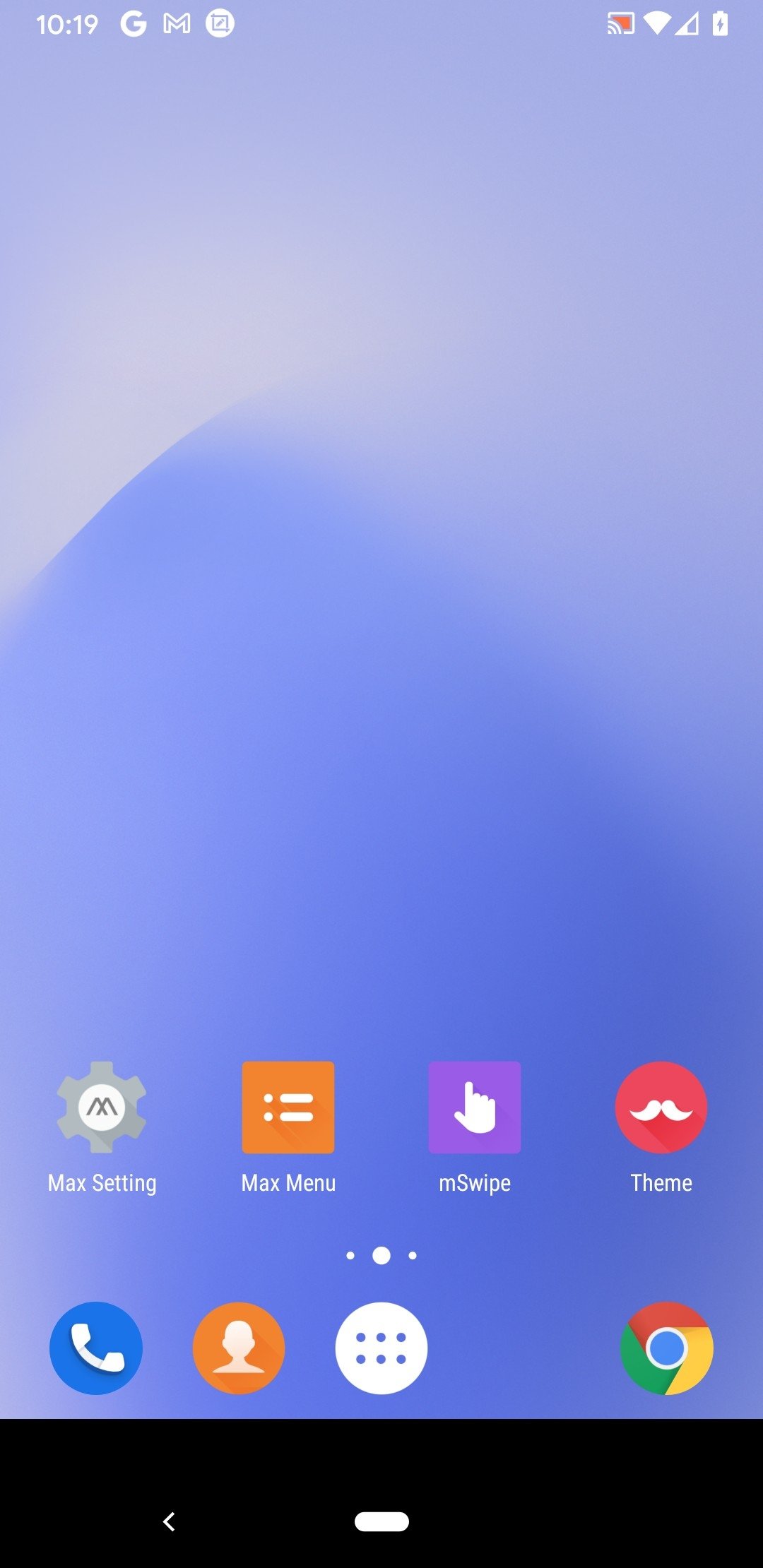In the top left corner, the screen displays the time "10:19," followed by a Google "G" icon, and then the Gmail icon with a small mail symbol. Adjacent to these icons, there is a circle containing a square and a checkmark. 

In the top right corner, a battery icon shows it is charging while the cellular signal is weak. However, the Wi-Fi signal is full, and there is also a Streamcast or streaming broadcast icon visible. 

The background is a gradient blend of bluish and purplish hues. 

Along the bottom of the screen, there is a gear icon labeled "Max Settings," followed by icons labeled "Max Menu," "Next Set and Swipe," and "Themes." The 
"Phone" and "Contacts" icons are also present, along with an icon consisting of multiple dots encircled in white. Near the right side, the "Google Chrome" icon is featured with its characteristic yellow, green, red, and blue design.

Additionally, there is a small pill-shaped icon at the bottom, and to its left, an arrow pointing left. The themed icons have distinctive features: the "Theme" icon includes a mustache, "Swipe" is represented by an index finger, "Max Menu" displays two horizontal eyes, and "Max Settings" is denoted by a gear with an "M" in the middle.